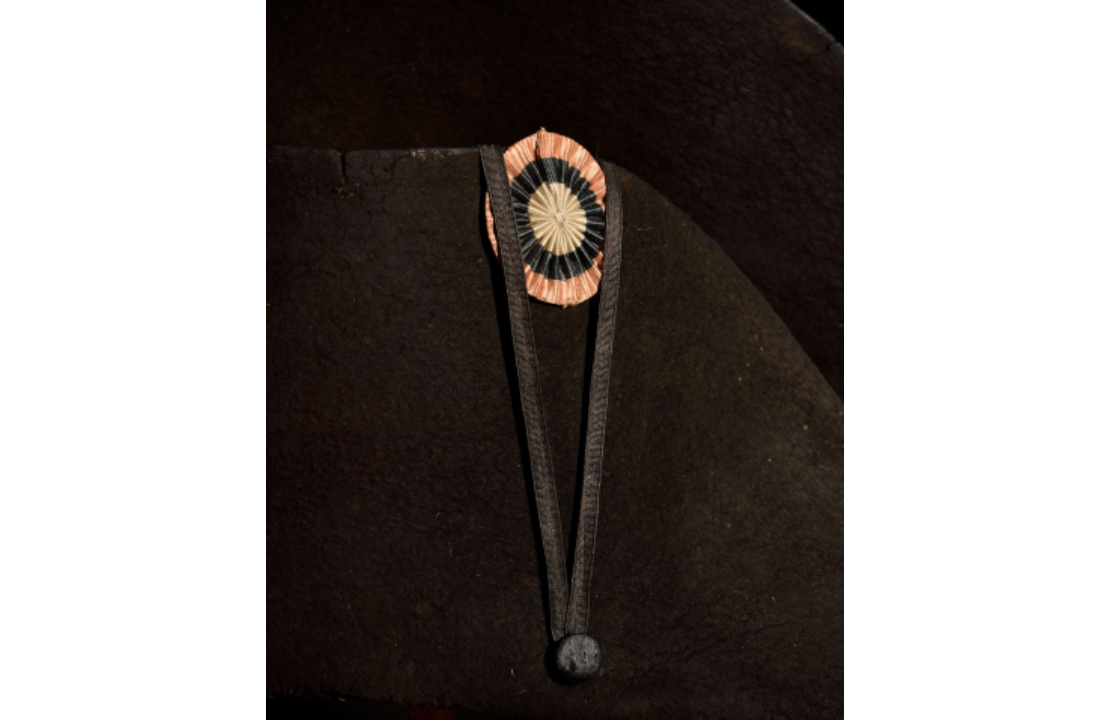The photograph is a detailed and zoomed-in image of a dark object, likely a military hat from an unspecified time period, possibly the 1700s. The background is composed of various shades of black and dark gray, with the upper portion of the image being almost entirely black. At the bottom of the photograph, there's a button from which a two-piece strap extends upward, widening as it moves towards the top. At the peak of the strap, there's a bullseye-shaped ribbon that secures it, consisting of concentric circles—white in the center, surrounded by a navy or black ring, and further encircled by an orange or reddish-pink ring. The circular ribbon bears a resemblance to an award or a medal, typically seen on military uniforms. Additionally, a cordage or trim, arranged in a V-shape, is visible, contributing to the overall intricacy of the object. The entire scene is quite dark, making it challenging to discern all details clearly.